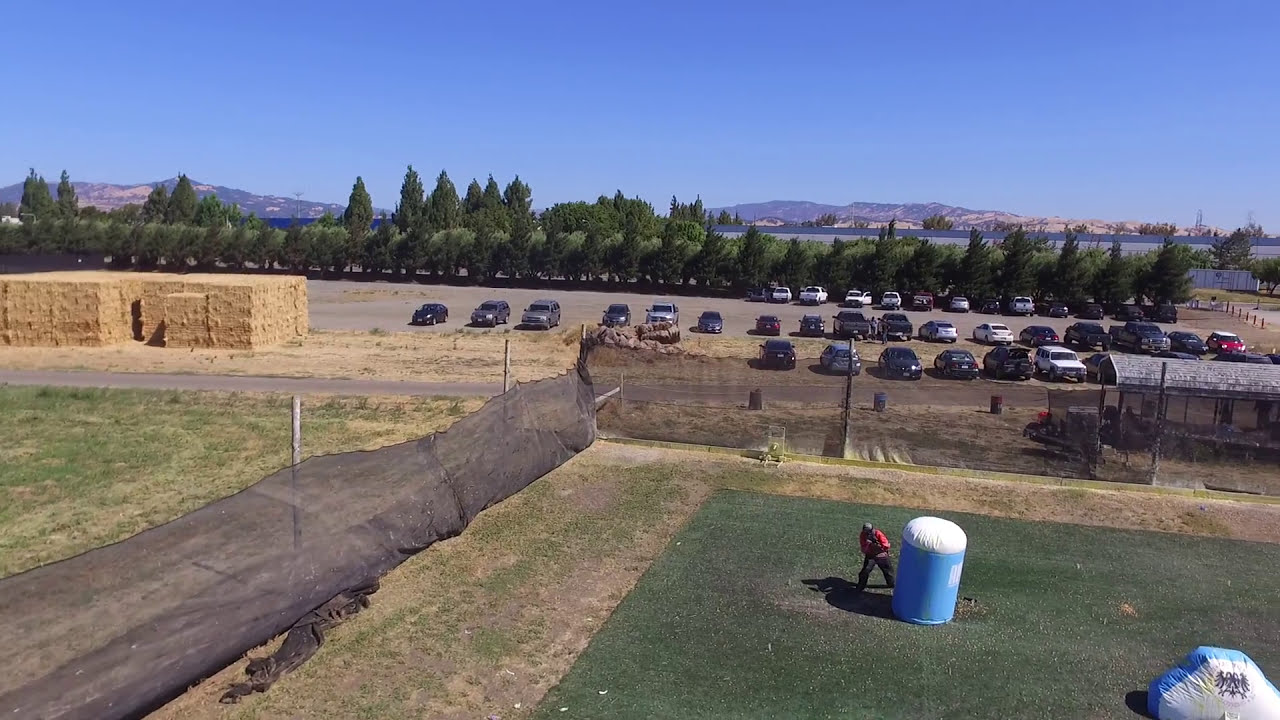This photo showcases a vibrant outdoor scene on a clear, sunny day with a striking blue sky. In the foreground, a man wearing a red shirt and black pants works behind a blue and white inflatable bunker on what appears to be a paintball field, which is fenced off with black netting. The field itself is covered in dark green sod or artificial grass. Off to the right, a blue, triangular inflatable can also be seen. 

Beyond the field, a large parking lot is filled with several cars and trucks, and to the left, stacks of hay bales are neatly piled. Further in the background, a line of tall pine trees stretches across the scene, with a gray building’s black roof peeking through. In the distance, majestic mountains rise against the azure sky, adding a touch of grandeur to the landscape.